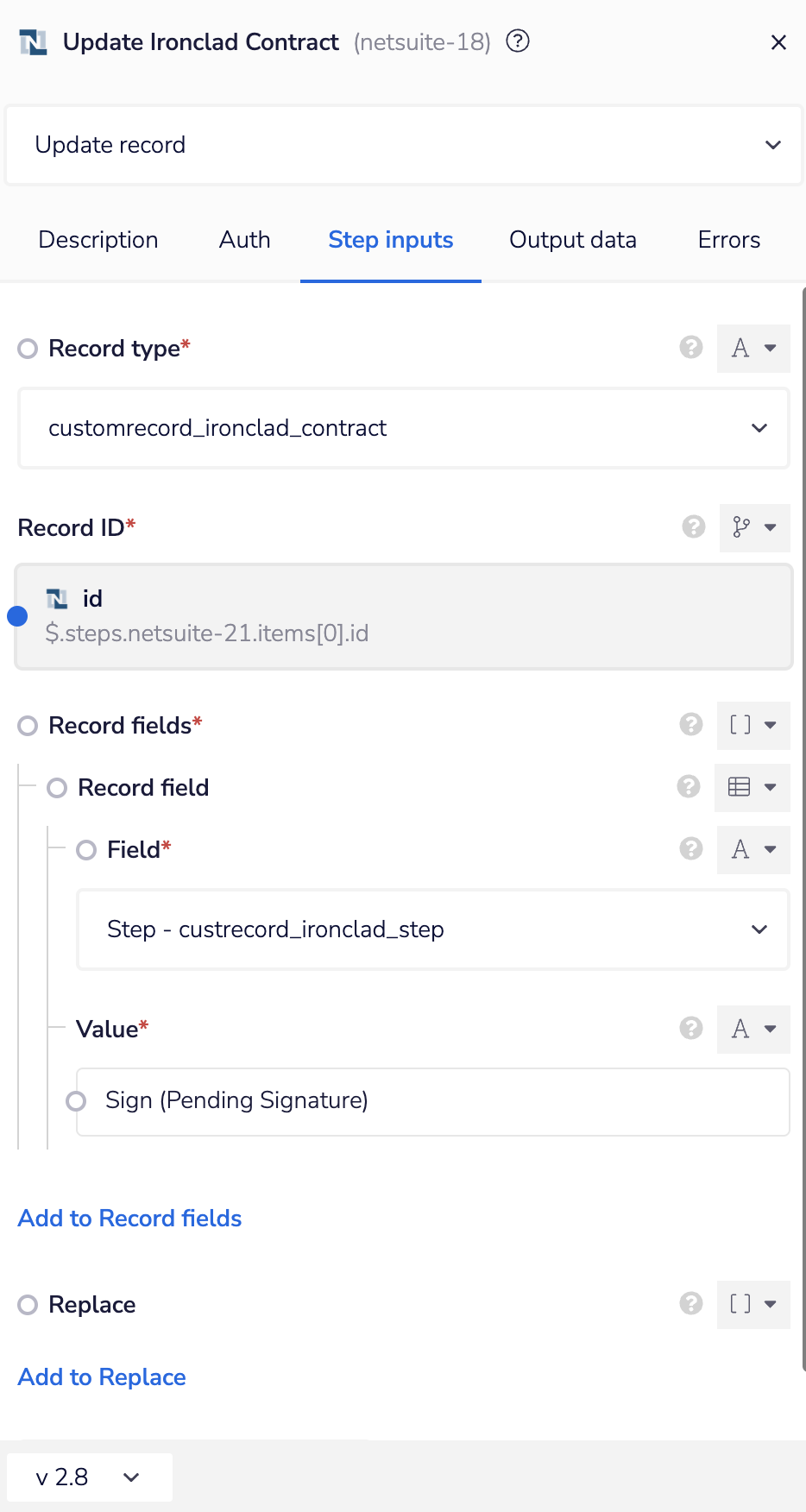**Caption:**

The image features a user interface on a white background for updating an RN-CLI contract. Key elements include:

- The title "Update RN-CLI Contract" prominently displayed in black.
- A deadline "Next July 18" and the mention of "NET Suite" (stylized as N-E-T-S-U-I-T-E) are visible. 

In the center-left, there is a circle containing a question mark and an X symbol, accompanied by the text "Update Record Description"—possibly indicating a help or error message.

On the left side, details like "Author" abbreviated as "A-U-T-H" are shown, along with step-by-step inputs labeled in blue, output data, and error notifications.

Several form inputs have red asterisks, denoting required fields:
- "Record Type" is next to a gray rectangle labeled "A".
- "Custom Record_ironclad_contract" displays as the field type.
- "Record ID" and its subsequent ID information are marked with a star.

Further fields contain:
- "Record Field" with a red asterisk.
- "Field," and "Value," which also have red asterisks.
- "Sign," with an annotation "(Pending Signature)."

Buttons for actions include:
- "Add to Record Fields" and "Replace," both highlighted in blue.
- Another blue action labeled "Add to Replace."

Each segment is marked clearly, ensuring users understand the importance of filling in necessary data before proceeding.